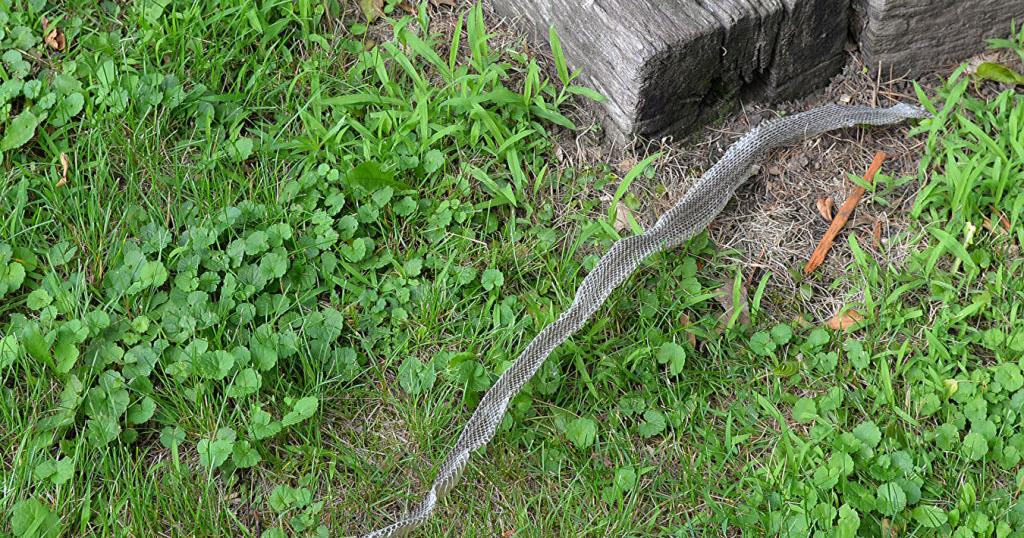The photograph captures a somewhat wild yard or lawn scene. Down on the ground, there is a mix of green grass, patches of weeds, and clusters of plants resembling clover, but with distinct leaf shapes. Scattered among the greenery are a few dead leaves and patches of dirt. Dominating the center of the image lies a very long, silvery-gray, translucent snakeskin, stretching out in a fairly straight line. The snakeskin's scale pattern is clearly visible. In the upper portion of the image, there is a dark area suggestive of a wall or a shadowed step. Adjacent to the snake's shed skin is a wooden structure, possibly a step or a piece of timber, with an additional wooden plank visible in the upper right corner. Adding a touch of color, an indistinct orange object lies near the snakeskin, perhaps a piece of cloth or a strap.